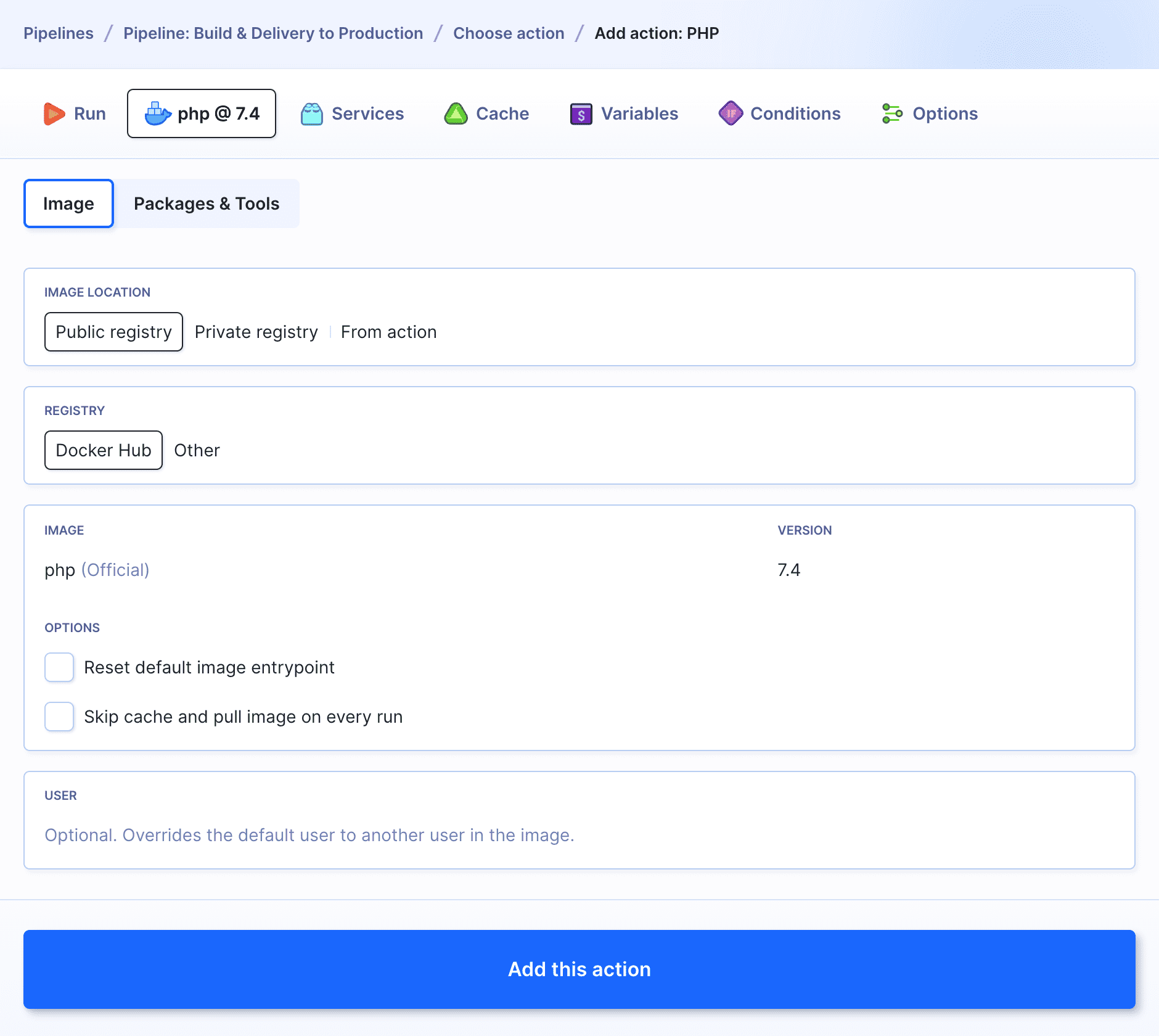The image is a screenshot of a web interface, seemingly from a DevOps or CI/CD platform. At the top left, the navigation bar features tabs labeled "Pipelines," "Pipeline," "Build and Delivery to Production," "Choose Action," and "Add Action PHP," with "Add Action PHP" darkened to indicate the current selection.

Below the navigation, there are several actionable buttons. The first-row buttons include "Run" and "PHP 7.4." Following this row are options labeled "Services," "Cache," "Variables," "Conditions," and "Options," each accompanied by a small icon.

Further down, another row presents "Images," "Packages," and "Tools," with "PHP 7.4" and "Image" highlighted. Below this, there's a section titled "Image Location" with three selectable options: "Public Registry," "Private Registry," and "From Action," where "Public Registry" is currently highlighted.

Next, under the "Registry" section, options include "Docker Hub" and "Other," with "Docker Hub" highlighted. Directly below, in the "Image" section, "PHP Official" is displayed with "7.4" under the "Version" label.

Under the "Options" heading, there are checkboxes—though unchecked—for "Reset Default Image Entry Point," "Skip Cache," and "Pull Image on Every Run." The final section, titled "User (Optional)," offers an explanation: "Overrides the Default User to Another User in the Image."

At the bottom of the screenshot is a prominent horizontal blue button with white text that reads "Add This Action."

This detailed caption incorporates all described elements and organizes them logically for clarity.